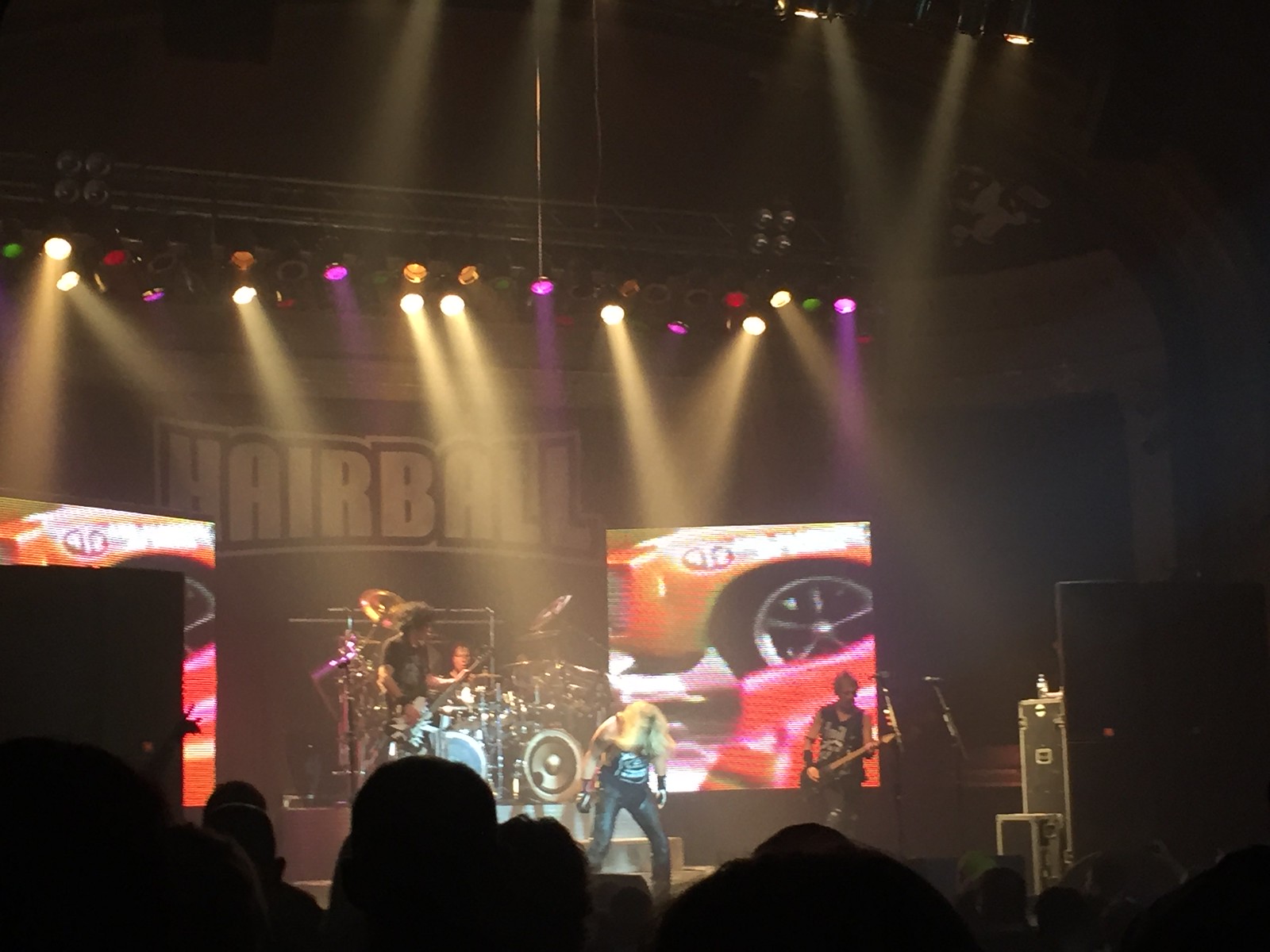The image is an indoor shot of a rock or metal band named "Hairball" performing live on stage. The stage is illuminated by a vibrant array of spotlights—pink, white, gold, red, and green—shining down on the band members. The band, consisting of around five members, includes a lead singer, a guitarist, a bassist, and a drummer. At the back of the stage, the name "Hairball" is prominently displayed in wide, bold white text. Flanking the stage are images of red sports cars, though one is partly obstructed by a speaker. The audience is visible as dark silhouettes in the foreground, indicating a lively and engaged crowd. The atmosphere is electric, with the band in full action amidst the dazzling lights and booming speakers, encapsulating the essence of a high-energy rock concert.